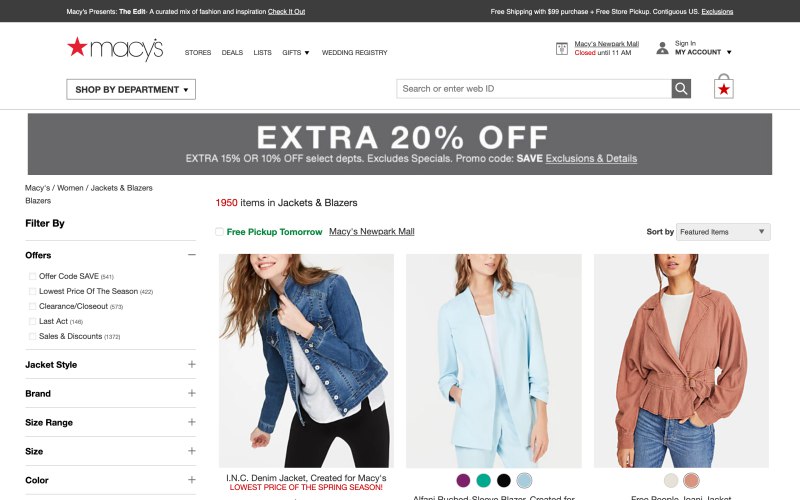This is a detailed screenshot of the Macy's website. At the top, there's a notification bar highlighting perks such as "Free Shipping" and "Macy's Presents." Below this notification is a thin grey bar, followed by a prominent white main menu bar featuring the Macy's iconic red star logo on the left. Adjacent to the logo is a dropdown option labeled "Shop by Department." The main navigation menu includes items such as "Stores," "Deals," "Lists," "Gifts" (with a dropdown), and "Wedding Registry." To the right, there is an alert indicating the closure of a mall location, alongside a "Sign In" option for account access.

Beneath the main navigation is a search field, followed by a shopping bag icon featuring a red star. Below this, a large grey alert bar dominates the screen, displaying a promotional message in bold white letters: "Extra 20% Off, Earn 15% or 10% Off Select Departments." The message further specifies that some specials are excluded and provides a promo code ("SAVE") with a link to exclusions and details.

On the left side of the page, there is a navigation menu focusing on Macy's women's jackets and blazers. This menu allows filtering by offers, jacket style, brand, size range, size, and color. On the right side, it indicates that there are 1,950 items available in jackets and blazers. Three images of women modeling different jackets are prominently displayed: a jean jacket, a light blue blazer, and a brown jacket. Though their eyes are not visible, the rest of their faces down to their thighs are shown, with color options for each item displayed below the images.